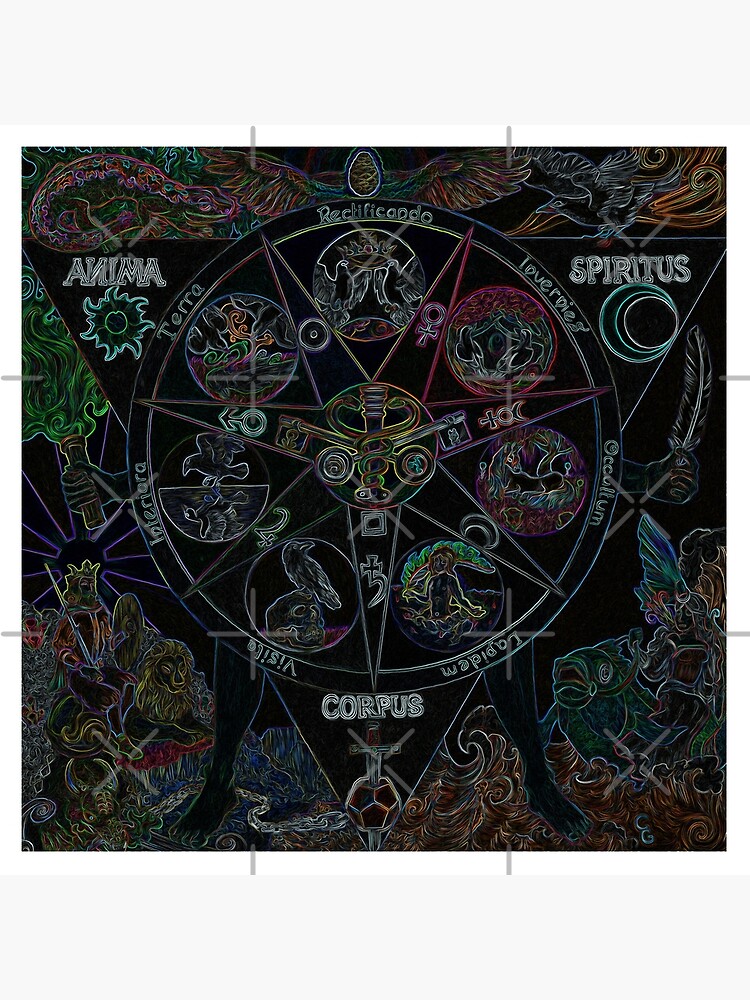The artwork is a detailed and intricate astrological or mystical chart, likely rendered in a medium resembling chalk on a black background. Central to the composition is a circle divided into seven spokes by a star with thin points and an encompassing triangle that frames the star. At the very core, there's a striking depiction of two serpents coiling around a dagger. Flanking this central motif, on the left and right, are images of two keys. Each of the seven sections created by the star and spokes houses different zodiac signs. Between these spokes are vibrant images and various symbols that might represent deities or mystical figures, colored in red, yellow, green, and dark blue hues. Surrounding these central figures are intricate decorations, adding to the sense of an elaborate astrological map. Notably, certain sections contain text, not in English but seemingly in Latin or a Romance language, with terms like "rectificado," "terra," and "oculum." Additionally, the artwork features a triangular perimeter; at the base of each inward-pointing triangle, a skeletal face of an animal with large, round eyes, a snout, and an open mouth can be seen. The upper-left and upper-right corners depict the sun with the text "ANIMA" and concentric circles with the text "SPIRUUS" respectively, while the bottom corner showcases a white triangle with the text "CORPUB." This composition weaves together elements from both real-world and fantastical astrology, creating a visually captivating and richly symbolic piece.